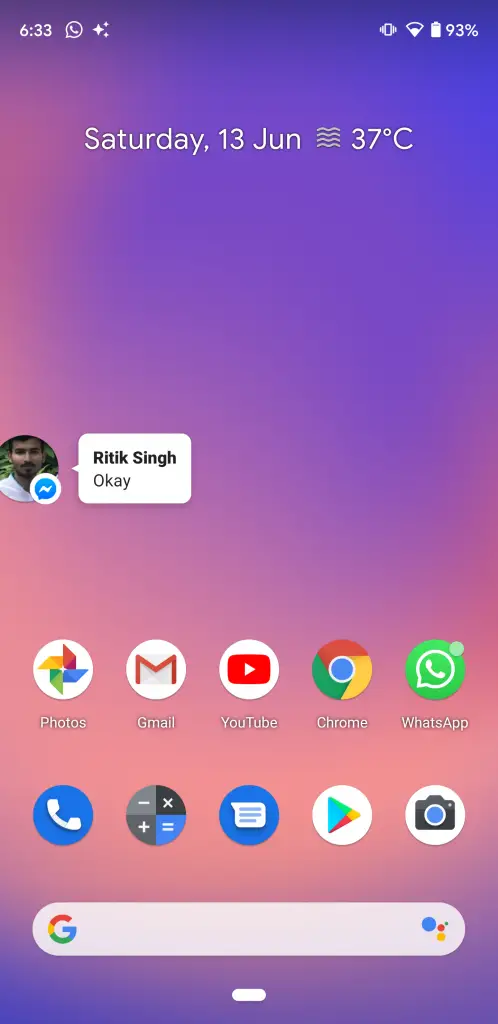A screenshot of a smartphone taken on Saturday, June 13th shows a vibrant display with a gradient background that transitions from a purplish hue at the top, blending into pink in the middle, and returning to purple at the bottom. The temperature displayed is 37°C. The phone screen is open to a messaging app, with a message from Ritka Singh that simply reads "okay." 

The phone's home screen includes several apps: Photos, Google Photos, Gmail, YouTube, Google Chrome, WhatsApp, and a Phone app. There’s another circular app icon with quadrants in shades of gray and blue, marked with math symbols such as minus, multiply, equals, and plus, likely a calculator app. Additionally, there is an unidentified app that seems to be a word processing tool, alongside the Camera app. At the bottom, there is a Google search bar, ready for input.